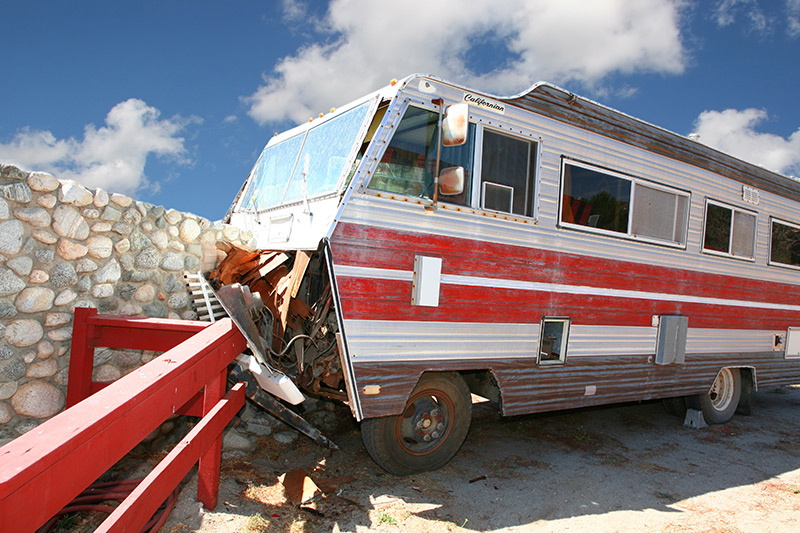In the photograph, we see an older, mostly red and white trailer that distinctly resembles a large camper or recreational vehicle. It is positioned towards the viewer’s left and has crashed into a red wooden fence and a cobblestone wall. The front of the trailer is severely damaged, appearing busted open, as if it might have torn off upon impact. The trailer features a faded paint job with red stripes running down the middle, bordered by small white pinstripes, and larger white stripes below, finished with a brown stripe at the bottom. The exterior seems to be constructed of metal, giving it a somewhat ridged, aluminum siding appearance.

There are multiple closed windows along the side of the trailer, which slide open sideways, and just above the driver's side window, there's a small badge labeled "Californian." Two rearview mirrors are visible on the driver’s side. The image captures a sunny day, with a blue sky dotted with a few clouds that do not obscure the bright sunlight, casting shadows of the trailer. The RV is stabilized with a block underneath one of its tires, though despite this, the entire front portion appears to be falling out. The scene is framed with a stone wall approximately five to six feet tall behind the trailer, adding to the sense of an unfortunate accident site.